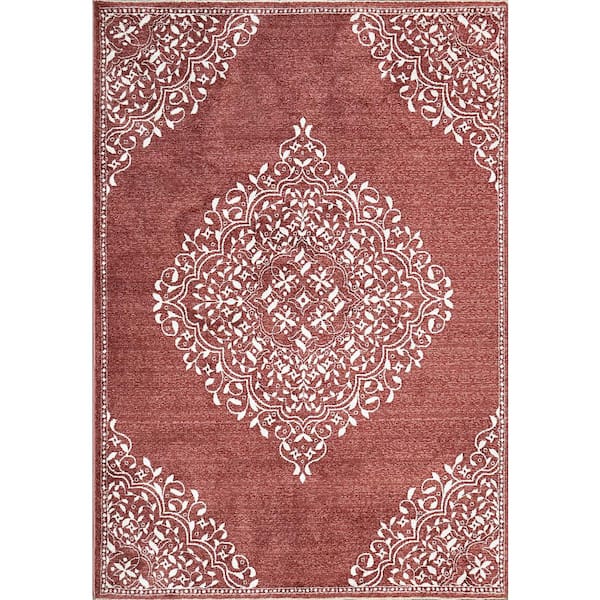This image depicts a small, Egyptian-style rug with a soft, rusty red background that has highlights throughout, giving it a textured fabric look. Around the edges of this rug runs a narrow, intricate white border. Each corner of the rug features a detailed, lacy white design reminiscent of leaves or a filigree, each scalloped pattern stretching down towards the center. The middle of the rug showcases a prominent diamond shape made from the same delicate white lace, mirroring the leaf-like designs found within the corners. Overall, the rug presents a blend of elegant craftsmanship with its repeating patterns and graceful symmetry, centered around the eye-catching diamond motif.